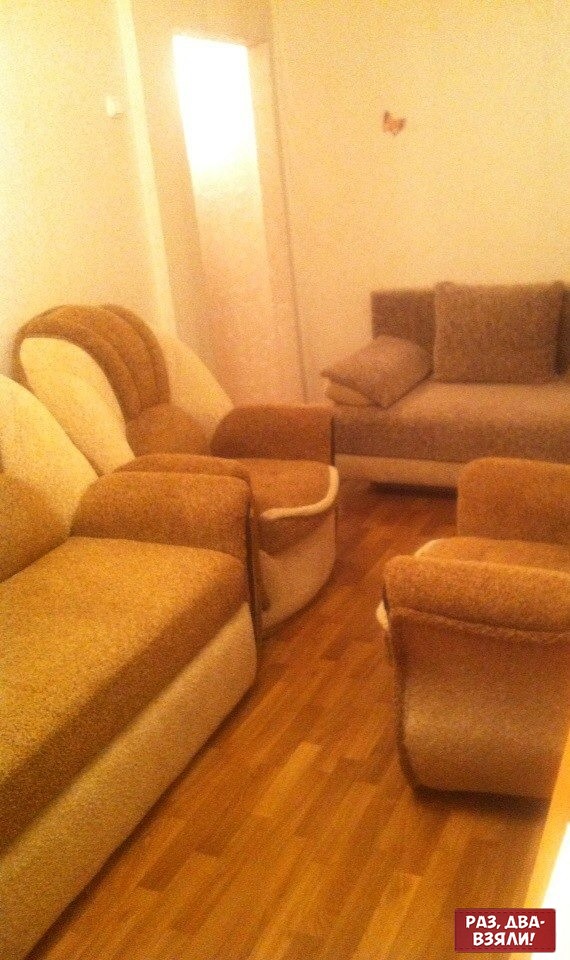The image showcases a uniquely styled, slightly blurry living room set with a portrait orientation. The scene is cast in a yellowish hue, likely due to lighting or a filter. At the center, there's a focal point of several brown couches, one notably resembling the shape of a dog. They feature a tweed-like material, with a combination of brown and white trim – brown seating areas and armrests with white accents at the back. Surrounding these larger, multi-person couches are matching single-person chairs. The room's backdrop includes yellow walls adorned with miscellaneous items, and a wooden floor, all contributing to a warm, eclectic atmosphere.